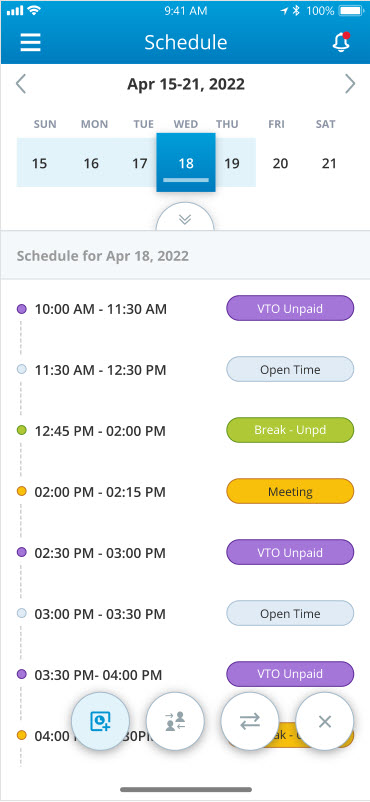Here's a detailed and cleaned-up caption for the image:

"Displayed is a person's weekly schedule for April 15th through the 21st, 2022. The current day, Wednesday, April 18th, is highlighted in dark teal. The specific schedule for April 18th, 2022, is detailed as follows:

- 10:00 AM to 11:30 AM: VTO (Voluntary Time Off) - Unpaid
- 11:30 AM to 12:30 PM: Open Time
- 12:45 PM to 2:00 PM: Unpaid Break
- 2:00 PM to 2:15 PM: Meeting
- 2:30 PM to 3:00 PM: VTO - Unpaid
- 3:00 PM to 3:30 PM: Open Time
- 3:30 PM to 4:00 PM: VTO - Unpaid

The bottom of the schedule has several icons which include:
- A person with an arrow going to the right
- Another person with an arrow going left
- Arrows pointing left and right
- An axe
- A box with what appears to be a camera, highlighted in blue

From 4:00 PM to 4:30 PM, the schedule might indicate an unpaid break, though the symbols on top make it difficult to confirm."